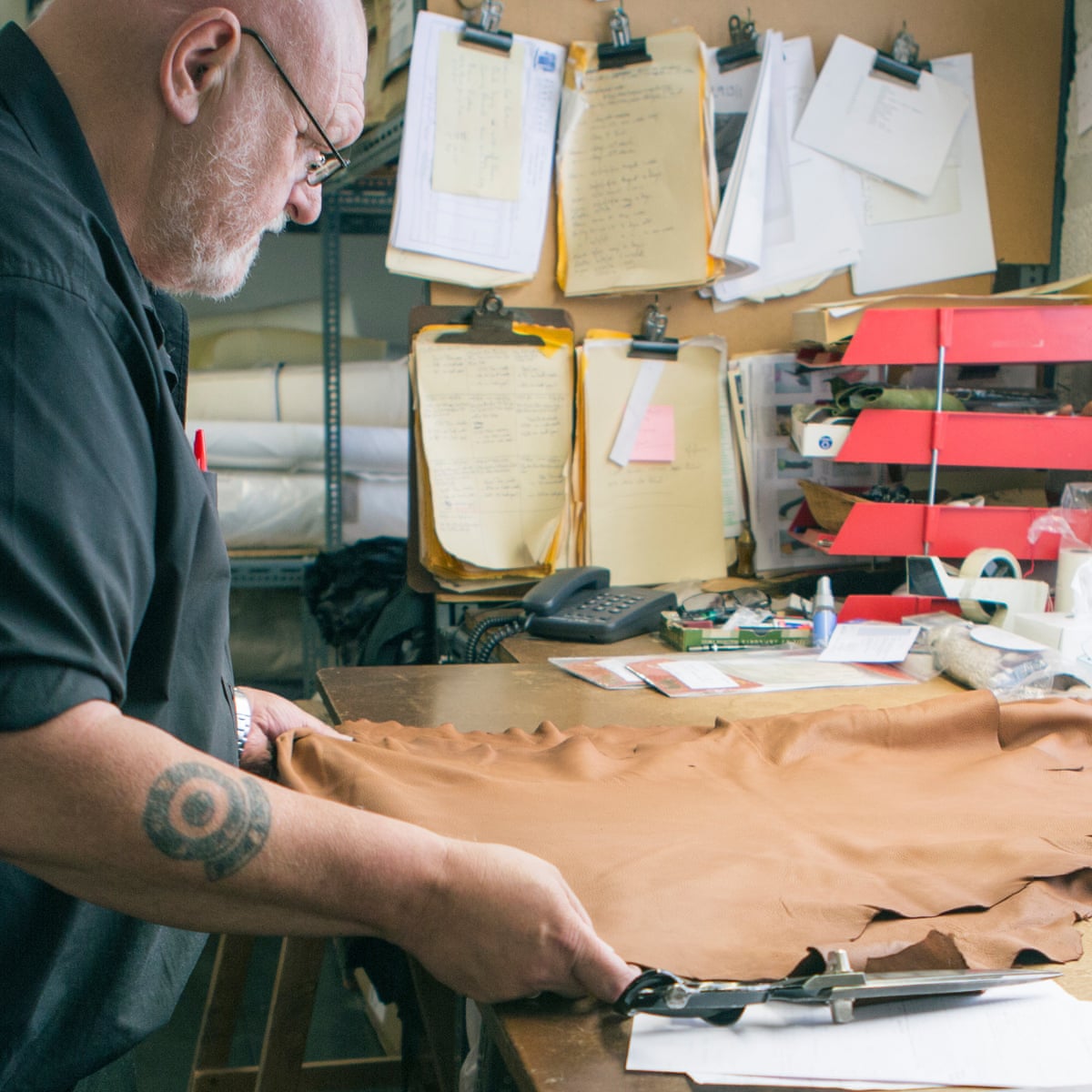The image displays a bearded, older man with a patchy white beard and black thin-frame glasses, situated on the left side, facing right. He is working intently on a piece of tan-colored, rippled fabric atop a wooden surface. A tattoo featuring a circle surrounded by another circle and an arch adorns his arm as he handles a pair of scissors. Clad in a black button-up shirt and an apron, with a red pen in his pocket, he appears to be engaged in a meticulous task, possibly measuring or tailoring. In the background, a corkboard with six clips holds multiple papers, hinting at detailed instructions or plans. To the middle-right, a spiral-wired dark gray phone rests on the table, surrounded by other work essentials such as pencils, with red shelves containing various items in the vicinity, suggesting a busy, well-organized workspace.